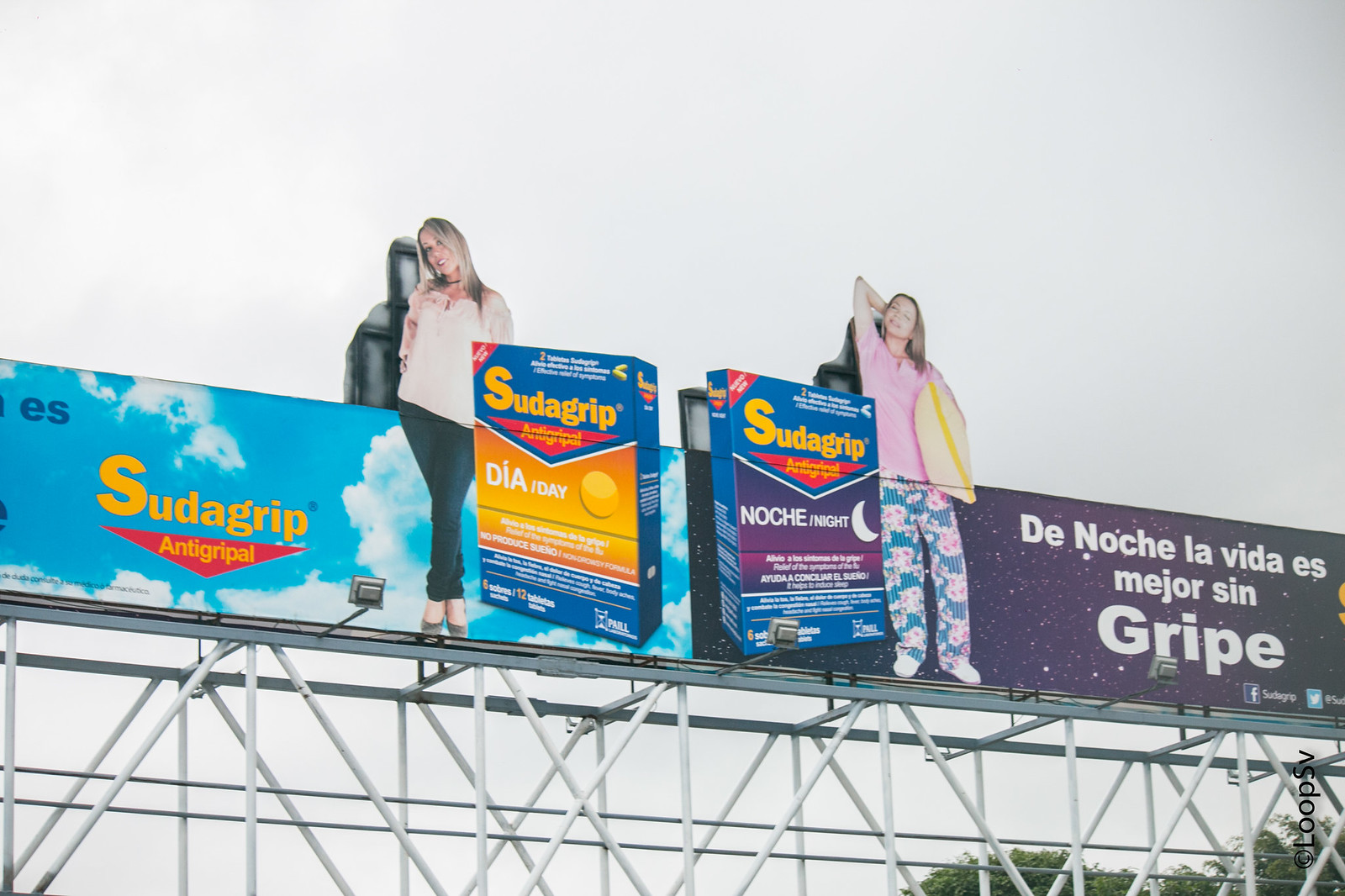The photograph captures an outdoor scene dominated by two adjacent billboards, both advertising "Pseudogrip" products. The billboards are mounted on a robust scaffold constructed from white and silver metallic poles, arranged in a grid-like pattern of intersecting horizontal and diagonal lines for structural strength. The left billboard promotes the daytime Pseudogrip product, set against a vivid blue sky with white clouds. It features a woman standing with her torso extending above the billboard's rectangular frame, wearing a white top and green pants. The central imagery on this billboard includes a rectangular pseudogrip box with a yellow center and a blue bottom, emblazoned with yellow "pseudogrip" text and a sun icon.

The right billboard advertises the nighttime version of Pseudogrip and is backed by a purplish, dark navy sky sprinkled with star-like white specks. The woman on this billboard, also extending beyond the frame, wears a pink top and colorful pajamas adorned with pink flowers, and carries a yellow blanket over her shoulder. The central image here is a similar rectangular pseudogrip box, but with a purple center and featuring a moon icon. The text on the billboards appears to be in Spanish, and the entire structure is set against a cloudy gray sky, with glimpses of green tree tops visible at the bottom right corner of the image. Additional smaller billboards can be seen in the background, contributing to the layered and detailed urban composition.